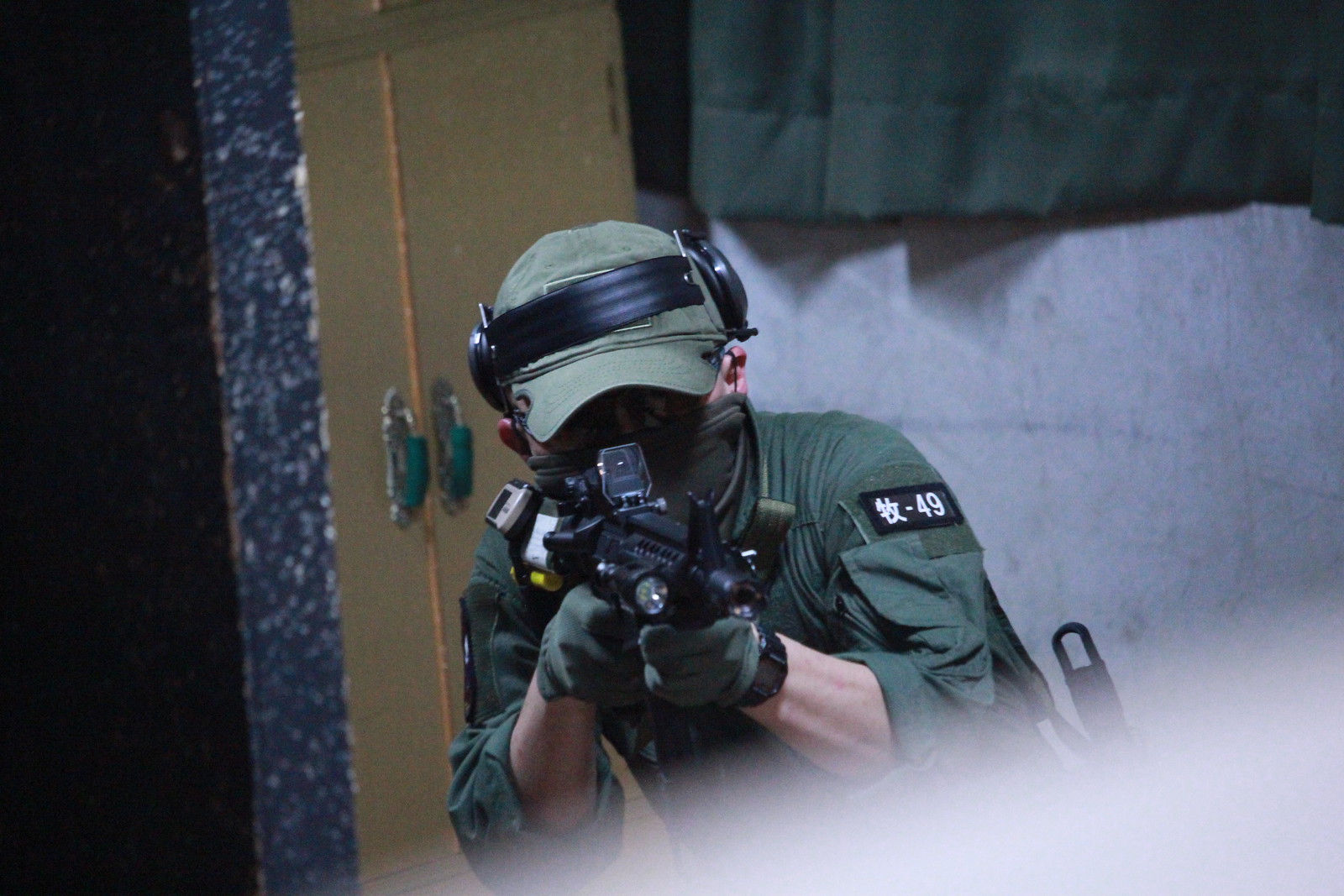The image depicts a man in a dark green, button-up shirt with a black patch displaying white writing, including an unrecognizable Asian character and the number "49." He is wearing a lighter green hat, black earmuffs positioned on top of his head, and green gloves. His face is obscured, and he appears to be aiming a black rifle equipped with a flashlight and sights slightly towards the camera, creating a potentially threatening perspective. Behind him, a gray cinder block wall is visible to his right, and to his left, there are what appear to be wooden cabinet doors with a blue strip on the side and black handles. A dark green curtain, similar in color to the man's outfit, is seen in the top right corner of the photo. The lower right corner of the image is partially blocked, possibly by the thumb of the person taking the picture. Additionally, the man is wearing glasses, and the general environment gives off an impression of an indoor setting, likely part of a building.